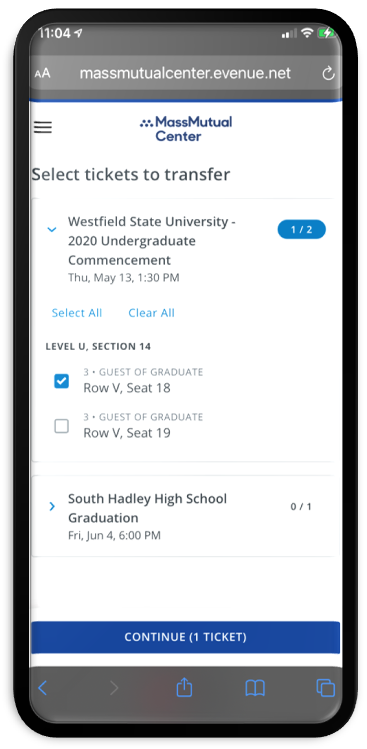The image is a detailed screenshot of a smartphone displaying a ticket transfer interface. The screen not only showcases the phone's display but also includes the phone's outline. At the top, the web address "massmutualcentre.evenue.net" is clearly visible. Below this, the interface prominently features "MassMutual Centre" with an option to select tickets for transfer.

Focusing on an event titled "Westfield State University 2020 Undergraduate Commencement," scheduled for Thursday, May 13th, at 1:30 PM, the page offers functionality to select or clear all tickets. The highlighted selection shows tickets for "3 guests of Graduate," specifying "Row 5, Seat 18" as checked, and "Row 5, Seat 19" as unchecked.

Below this detailed information, another event is listed: "South Hadley High School Graduation," which is set for Friday, June 4th, at 6:00 PM.

At the bottom of the screen, a prominent blue button with white text reads "Continue (1 ticket)," inviting the user to proceed with their selection.